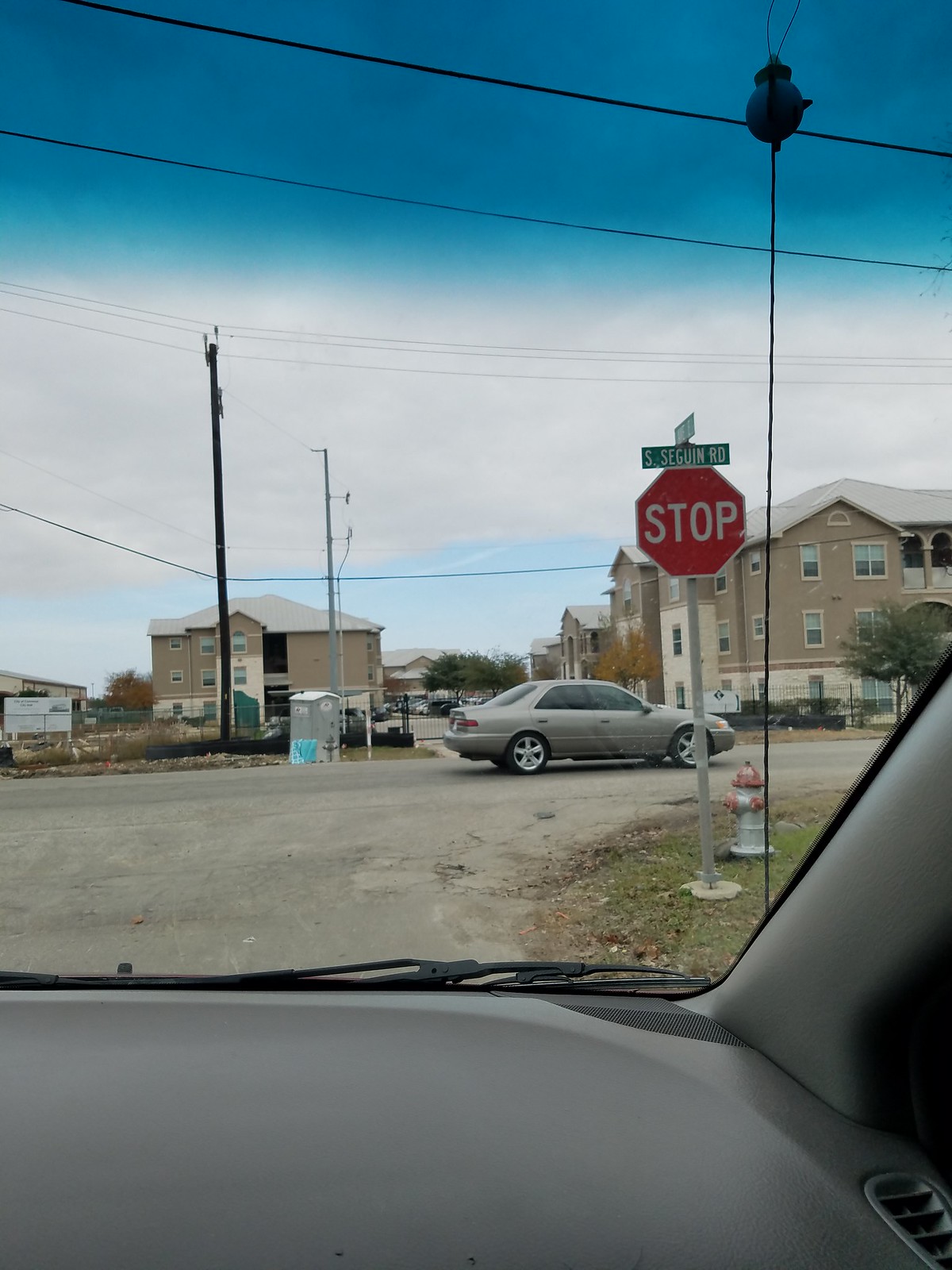The image, taken from inside a car, shows a detailed view of a neighborhood scene at a stop sign. The car's gray dashboard and the edge of the window frame the view, with a windshield wiper visible. Dominating the view is a large red stop sign, with a green street sign above it reading "South Seguin Road." Below the stop sign, there is a silver and red fire hydrant alongside a patch of green grass. The road ahead is dark black with a little bit of dirt, and a silver car is seen traveling to the right. In the distance, there is a construction site marked by a silver portable toilet and a large white sign, too distant to decipher. Surrounding the area, there is a fence and several power lines crisscrossing a blue sky filled with clouds. The background reveals a beige apartment complex with three-story buildings, each featuring balconies. These apartments stretch further back and are part of a gated community visible in the distance. Trees are scattered across the scene, emphasizing the neighborhood atmosphere.